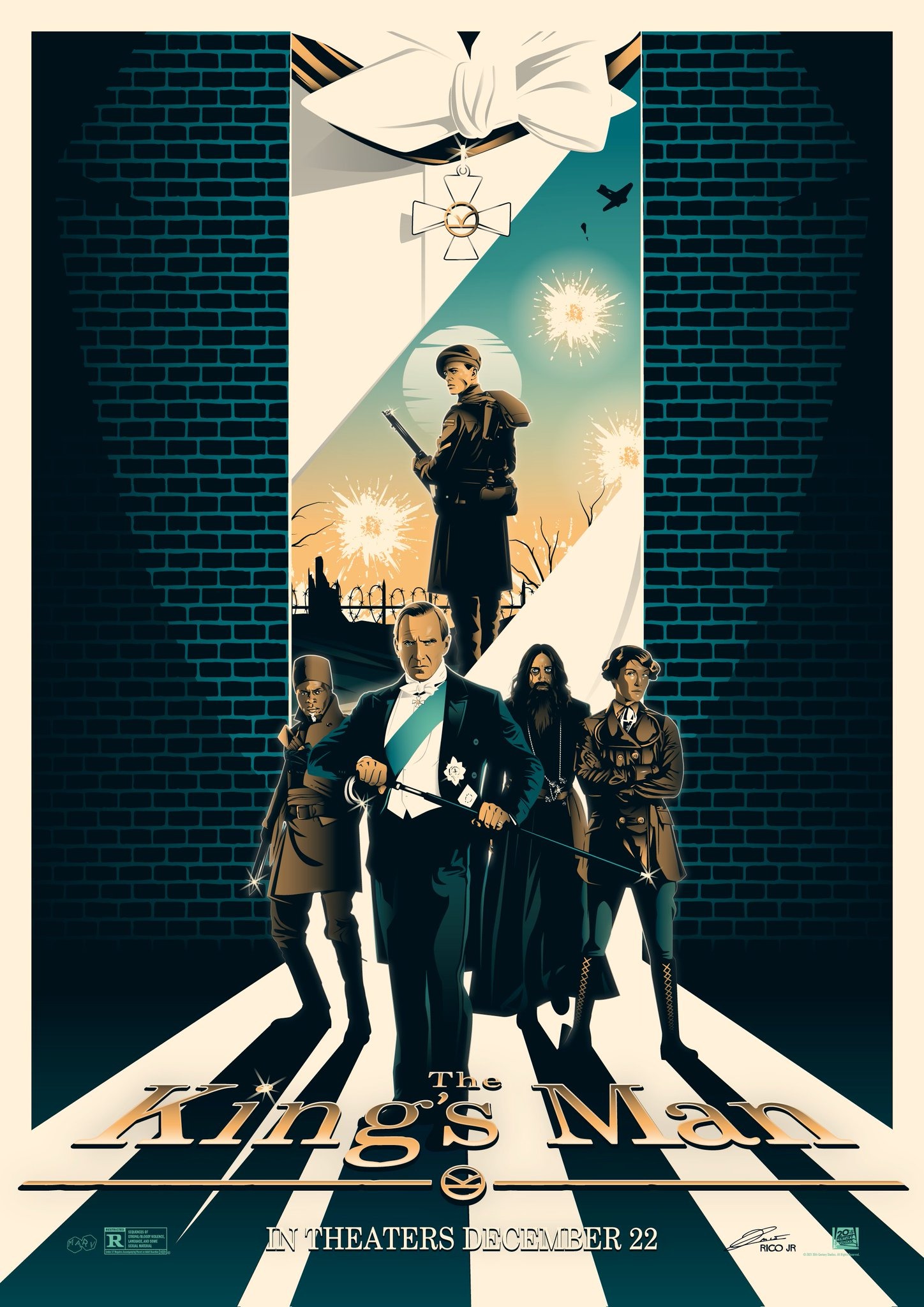In a vibrant, cartoonized movie poster for "The King's Man," an intricate background of black bricks with turquoise caulking provides a textured setting. Dominating the top center is an ornate white bowtie adorned with a dangling cross charm, contributing to the poster's sophisticated aesthetic. In the upper portion, a soldier from World War I, clad in an army green suit and beret, is seen holding a rifle and looking over his shoulder as explosions and fireworks illuminate the sky behind him. 

Central to the composition, four characters stand prominently. Foremost is a well-dressed man with hair parted to the left, wearing a white dress shirt, a tuxedo, and a teal sash across his chest. He is dramatically poised, pulling a sword from his cane and staring directly at the viewer. To his side, a man in a brown uniform also holds a spear, while a rugged individual with a beard and dark eyeliner stands nearby, dressed in a flowing gown. Completing the quartet is a woman with short hair, outfitted in a brown, double-breasted jacket, pants, and knee-high boots.

At the bottom of the poster, golden text reads "The King's Man," accompanied by details in white: "In Theaters, December 22nd." Additionally, the left corner bears an "R" rating, while the right corner features the text "Rico Jr." and "20th Century Fox," framing this immersive and detailed portrayal of the film's release.